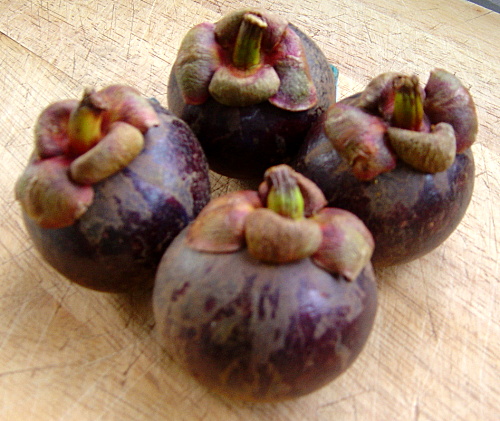A photograph showcases four purple fruits, each with brown mottling near the top where their dried leaves have receded. These fruits bear a resemblance to plums and feature green stems surrounded by four petal-like leaves. The fruits are slightly dirty and rest in a diamond pattern on a roughly finished, light brown wooden table. The image appears to be taken indoors, possibly in a kitchen, with the fruits positioned closely together, creating a cozy, clustered arrangement.